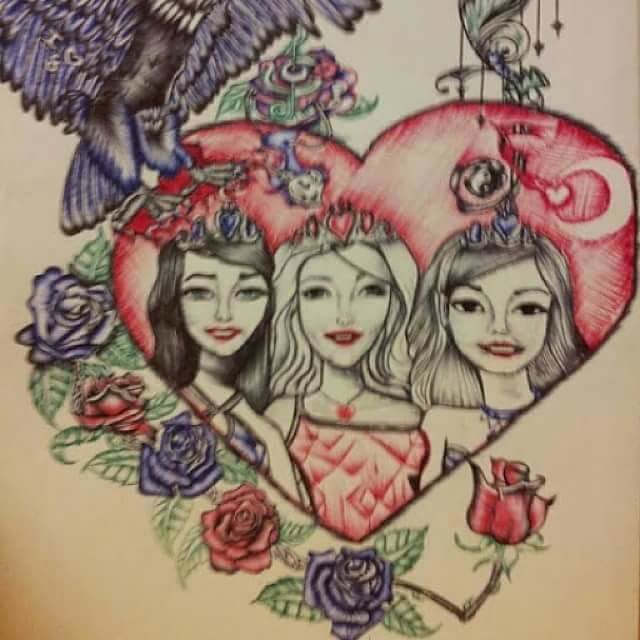The photograph depicts an intricately drawn and colored illustration, likely originating from an adult coloring book due to its sophisticated detail. The background is a pale grayish-peach hue. Dominating the center is a large heart with red edges that gradually blend into a light pink. Inside this heart are three crowned women. The central figure has long, white hair and wears a red crown. She is adorned with a pink dress and a necklace. Flanking her on either side are two other women—one with medium grayish hair and the other with dark hair. Both wear violet-blue crowns, matching dresses, and necklaces. All three women have fair skin and red lipstick.

Surrounding the left side of the heart are alternating roses in violet-blue and red. These flowers extend from the bottom left corner, up and around to the top right side. A single, unidentified drawing on the top left corner appears to resemble feathers, possibly from a bird. The artwork is rich in detail and color, making it a possible candidate for an adult coloring project.